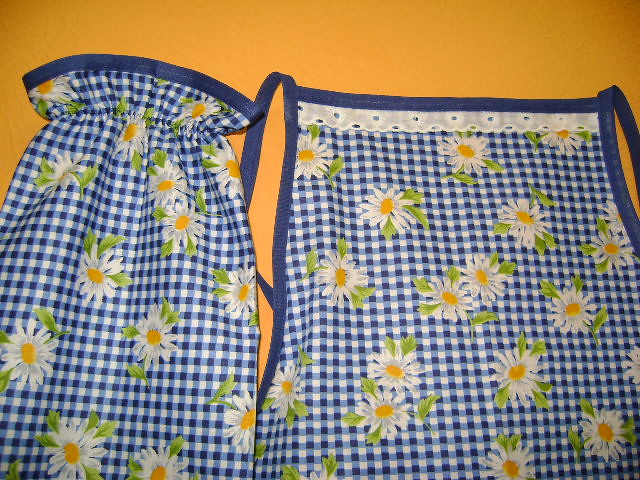This photograph features two aprons placed side-by-side on an orange surface, likely a table or countertop, and illuminated by even artificial lighting. Both aprons share a crisscross pattern of blue, light blue, and white stripes, resembling a basket weave or checkerboard design. Adorned with a repeated motif of daisy flowers—white petals, golden yellow centers, and green leaves—these aprons are nearly identical. However, the one on the right is distinguished by a white border at the top. One apron is scrunched up and tied, while the other lies flat and untied next to it, suggesting their use as kitchenware or cooking attire. The setting and lighting imply this could be a styled product image possibly aimed for a storefront display.